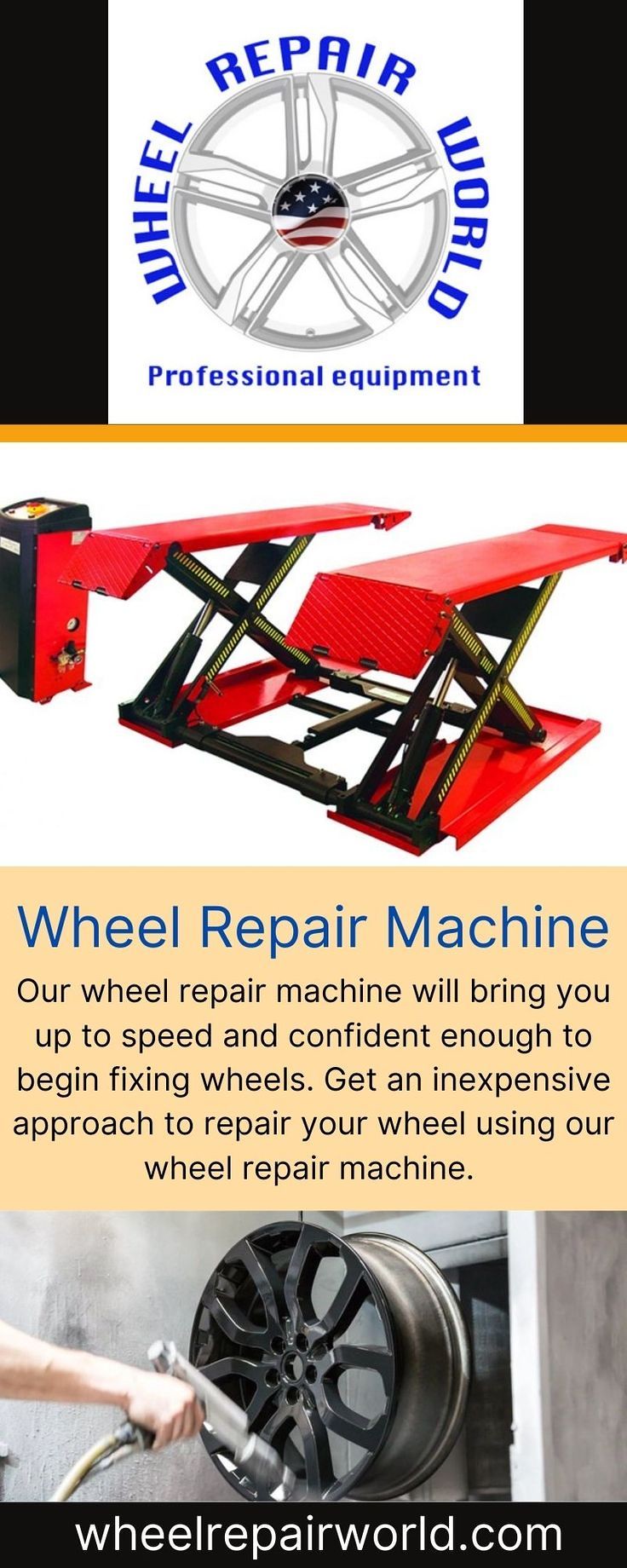An advertisement for a wheel repair machine is depicted in this image, structured into three sections against a predominantly white background. The top section, set against a black background with a yellow bottom border, features a chrome rim framed by blue text stating "Wheel Repair World," with a depiction of the American flag in the center. Below this, the words "Professional Equipment" are displayed in blue text.

The middle section showcases a piece of equipment resembling a car jack, featuring a red top, blue body, and black supports, accompanied by a control unit on the left. This section, set against a white background, presents the headline "Wheel Repair Machine" in large blue font, followed by the description: "Our wheel repair machine will bring you up to speed and confident enough to begin fixing wheels. Get an inexpensive approach to repair your wheel using our wheel repair machine." This section also includes an image of a black tire being brushed by someone.

The bottom section contains a black bar with the text "wheelrepairworld.com" written in white, concluding the ad. The entire layout is well-organized, with sections stacked vertically, visually clear, and easy to read. The background setting appears to be a workshop, consistent with the professional equipment theme.